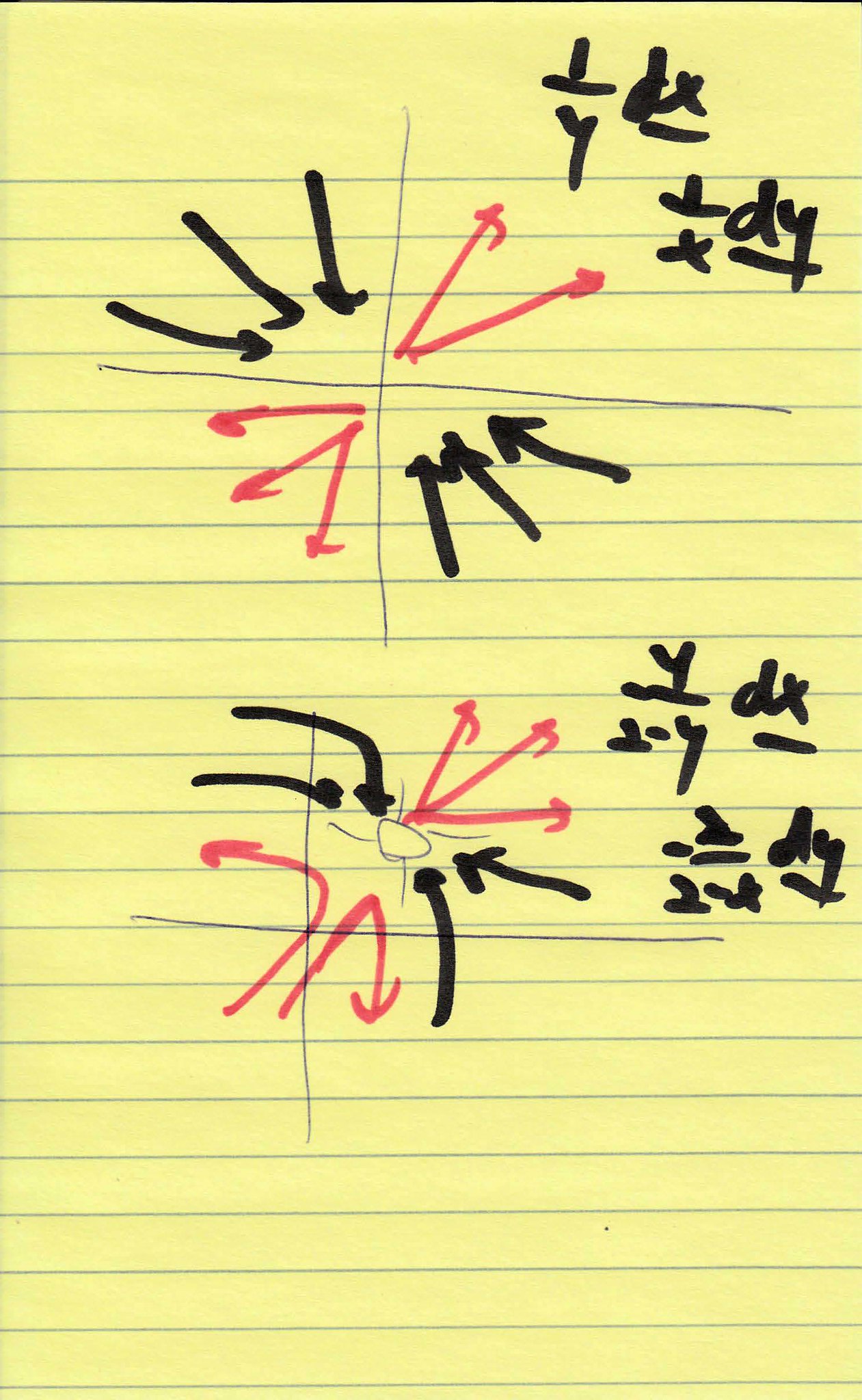This color photograph showcases a section of a yellow lined paper filled with various handwritten annotations, including arrows and mathematical equations. At the top of the image, a cross is prominently drawn, segmenting the sheet into four quadrants. Each quadrant features a set of three black arrows: the upper left and upper right quadrants have arrows pointing inward, while the lower left and lower right quadrants have arrows pointing outward. Additionally, in the upper right quadrant, there are two red arrows drawn with a heavy black marker, also pointing outward in the opposite direction to the black arrows.

Towards the top right corner of the image, handwritten equations are visible yet partially illegible. The notation includes "1/y" and "1/x dy." Below this, another set of annotations appears similar in structure, with a cross and corresponding arrows. Here, the lower half of the sheet continues with mathematical expressions, where "y/2 - y" and "dx" can be deciphered, and another equation at the bottom remains unreadable due to its faint visibility. The intricate details in the handwriting and the vibrant use of color contribute to a visually engaging and complex presentation of mathematical concepts and directional indicators.